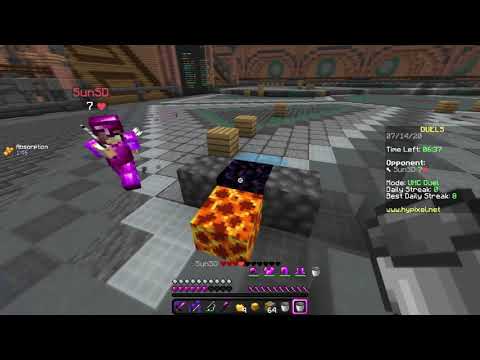This screenshot, captured from a video game on either a mobile device, console, or computer, vividly portrays a gaming interface with numerous details. A black border frames the top and bottom of the image, encapsulating a room with a patterned gray floor tile and walls adorned with various brown and green circular designs. Central to the image is a purple humanoid figure, reminiscent of a LEGO character or robot, identifiable by its faint facial features. Above the figure, the partially discernible text "S-u-n-s-d" appears, accompanied by a number "7" and a heart icon, implying a health indicator.

The game's interface is enriched with informational text and icons. The bottom of the screen displays a comprehensive bar featuring health, food, and item indicators, important for the player's status. Text on the image reads "duels, time left, opponent, mode, daily streak, best daily streak, www.hypixel.net," hinting at the game's mode and player progress. The floor, covered in varying gray square tiles, has several cubes, including gray, black, and an orange-yellow one, suggesting obstacles or interactive elements in the game.

Intricate details like small, illegible icons below the primary panels and additional writing on the right side in white, yellow, and green colors indicate dynamic in-game information. The room's visual intricacies, from its scattered yellow crates to the multicolored wall patterns, and the presence of text relaying player stats and game dynamics, collectively offer a comprehensive snapshot of this intricate gaming environment.